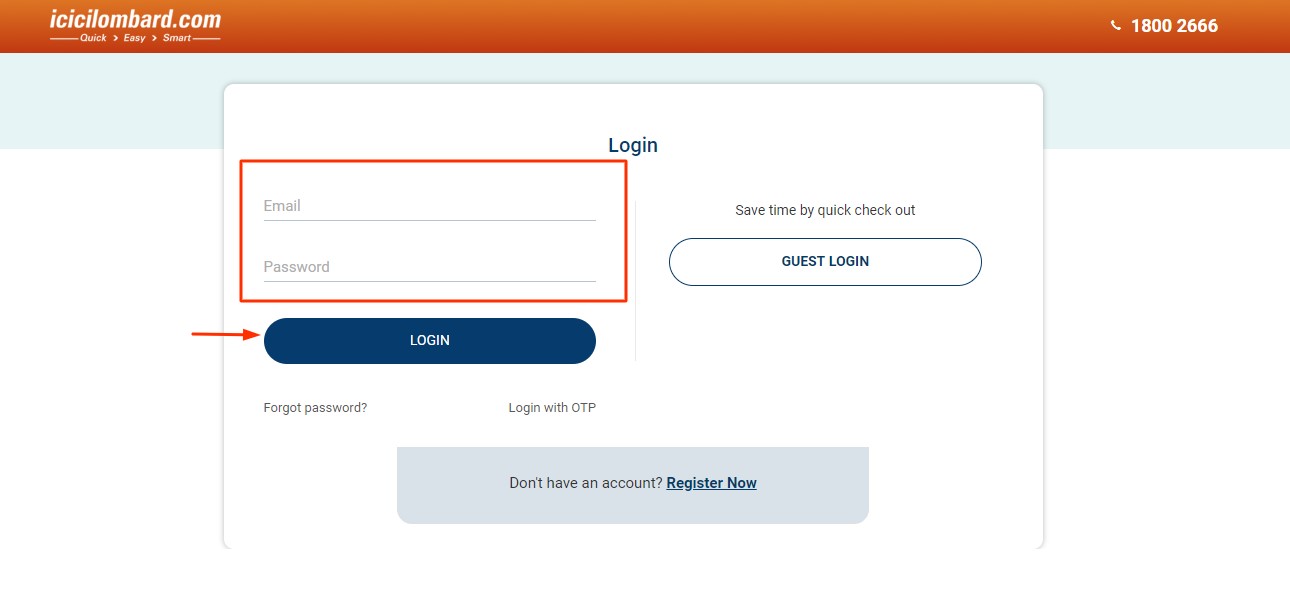This is a detailed screenshot of a website.

In the upper left corner, a bold red banner displays the text "ICCLombard.com" prominently. Beneath this, the words "Quick Easy Smart" are positioned. The upper right corner features a phone handset icon followed by an incomplete contact number, "1-800-2666."

Below this section, there is a horizontal gray bar. Central to the screen is a prominent white pop-up menu. At the top of the menu, the word "Login" is showcased in blue font. On the left side of the menu, there are two input fields, one labeled "Email" and the other labeled "Password," both circled in red for emphasis.

Beneath these fields, a blue oval button with white font reads "Login," accompanied by a red arrow pointing towards it. This setup appears to serve as a tutorial, presumably for users unfamiliar with the login process.

Further down, the options "Forgot Password" and "Login with OTP" are available. To the right, text advises, "Save time by Quick Checkout: Guest Login."